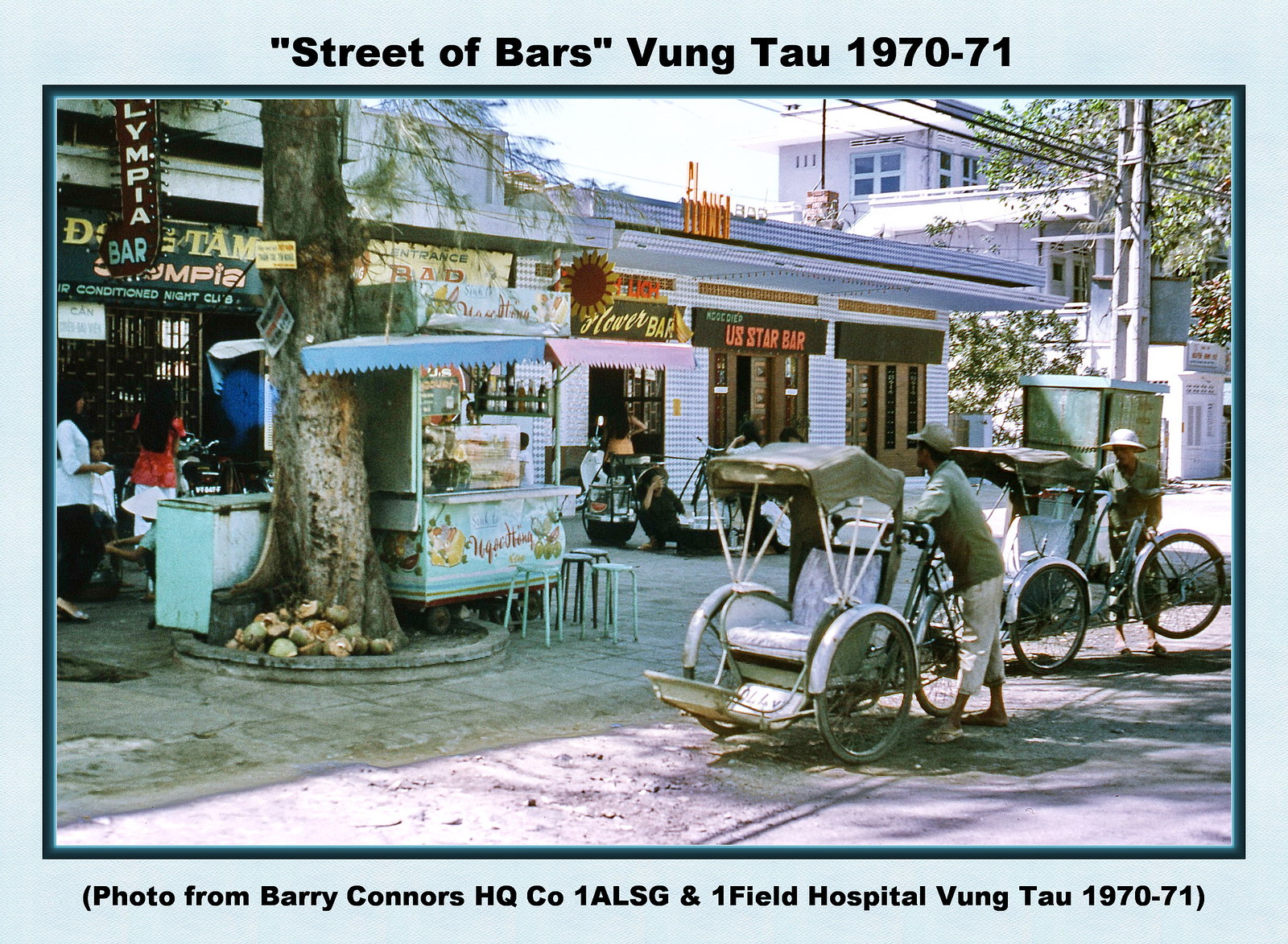The image is a historical photograph of a bustling street in Vung Tau, 1970-71, framed in light blue with captions at the top and bottom. At the top, it reads "Street of Bars, Vung Tau, 1970-71," and at the bottom, it notes "Photo from Barry Connors, HQ CO 1 ALSG, and One Field Hospital, Vung Tau, 1970-71." The scene captures a lively, unpaved street flanked by stone or clay sidewalks.

The street is lined with various small buildings and establishments, predominantly bars such as the Olympia Bar, US Star Bar, and Flower Bar, reflecting the street's nickname, "Street of Bars." In the background, pedestrians stroll along the sidewalk, while several street vendors and concession stands add to the vibrant street life. Notably, there is a tree with a small stand beside it, covered by a flat, umbrella-like canopy, possibly an ice cream stand with a small fridge or freezer.

Additionally, men in hats, possibly taxi or carriage drivers, wait beside their carts or buggies on the street, anticipating customers. The photograph's perspective, taken perpendicular to the street, provides a clear and detailed view of this dynamic urban scene from the Vietnam War era.